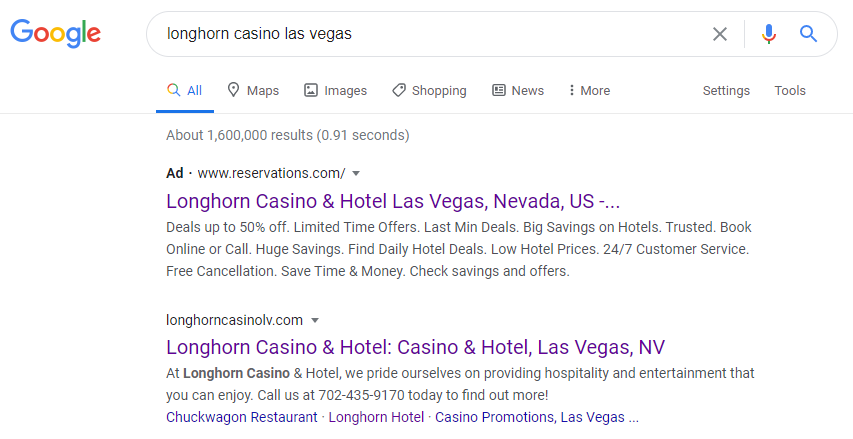This image captures a laptop screenshot in landscape mode with a predominantly white background. In the upper left corner, the Google icon is visible, adjacent to the search bar. The search bar contains the query "Longhorn Casino, Las Vegas," indicating that the user has typed this phrase to search for related information.

Below the search bar, there are several navigational tabs labeled "All," "Maps," "Images," "Shopping," "News," "More," "Settings," and "Tools." The "All" tab is highlighted in blue, suggesting it is currently active. A line of text below these tabs displays that approximately 1.6 million results have been found.

The first result shown is an advertisement from www.reservations.com, which directs to the Longhorn Casino and Hotel in Las Vegas, Nevada. This link appears in purple, indicating it has been visited before.

Following the advertisement, the second result is from longhorncasinolv.com, also addressing the Longhorn Casino and Hotel in Las Vegas, Nevada. Similarly, this link is in purple, signifying previous visitation by the user.

Beneath the main result headings on the second row, there are additional live links: "Chuck Wagon Restaurant," "Longhorn Hotel," and "Casino Promotion Las Vegas," each offering specific sections related to the Longhorn Casino. These links are also active, underlining the user's detailed exploration of information regarding the Longhorn Casino in Las Vegas.